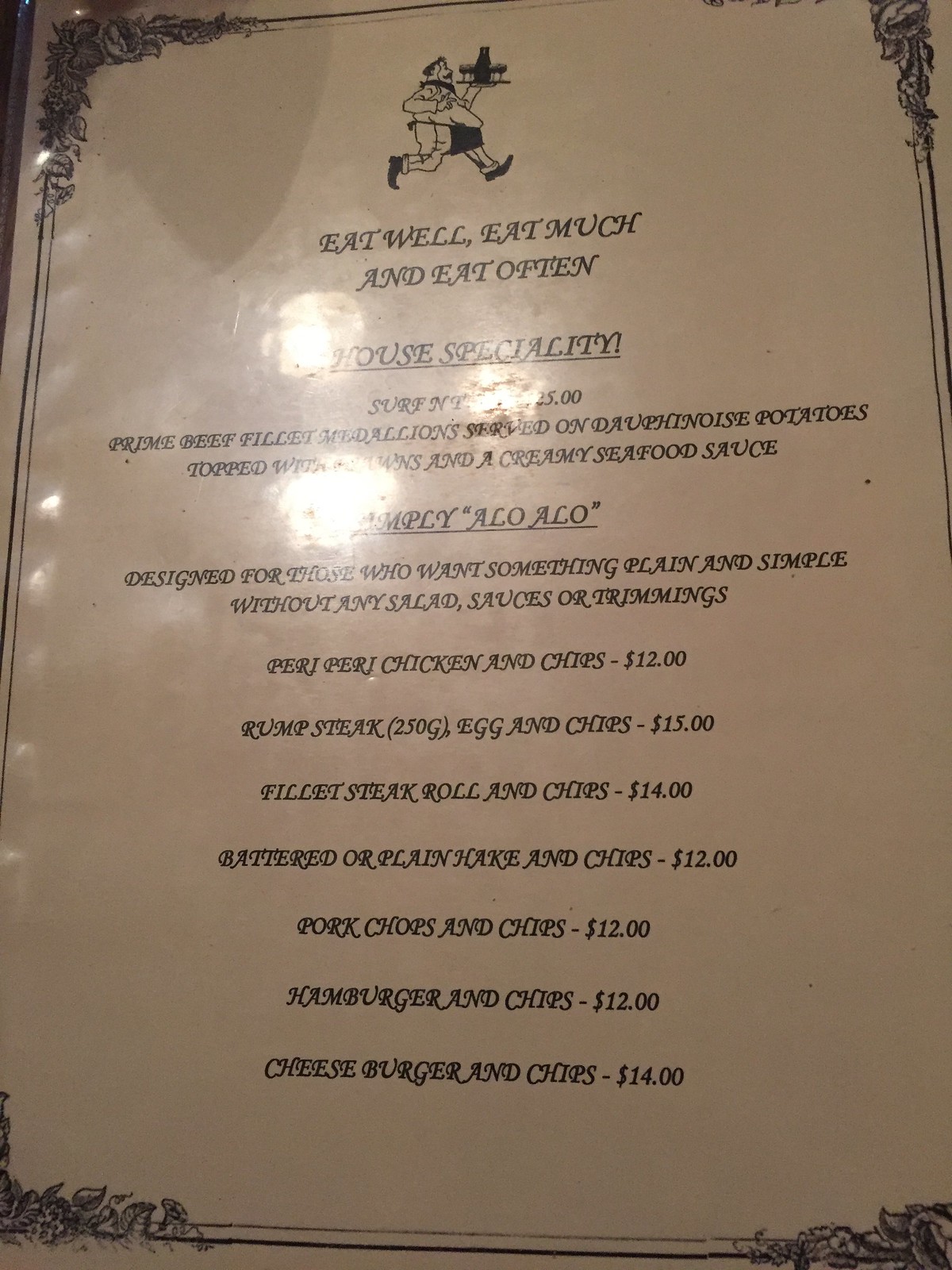This photograph showcases a laminated white restaurant menu, adorned with a delicate double-lined border featuring ornate foliage at the corners. At the top of the menu, a somewhat overweight waiter dressed in white attire, except for a dark apron, neckerchief, and shoes, is holding a tray with a bottle of wine and some wine glasses. 

The heading beneath the image, written in unattractive, all-capital calligraphy-like font, reads: "EAT WELL, EAT MUCH AND EAT OFTEN. HOUSE SPECIALTY!" The special mentioned is "Surf and Turf" (though partly obscured by glare from overhead lights) priced at $25, described as prime beef filet medallions served on dauphinoise potatoes topped with a creamy seafood sauce.

Following this, a section labeled "Alo Alo" offers options for those preferring plain and simple dishes without salad, sauces, or trimmings: 
- Peri-peri Chicken and Chips: $12
- Rump Steak, Egg, and Chips: $15
- Filet Steak Roll and Chips: $14
- Battered or Plain Hake and Chips: $12
- Pork Chops and Chips: $12
- Hamburger and Chips: $12
- Cheeseburger and Chips: $14